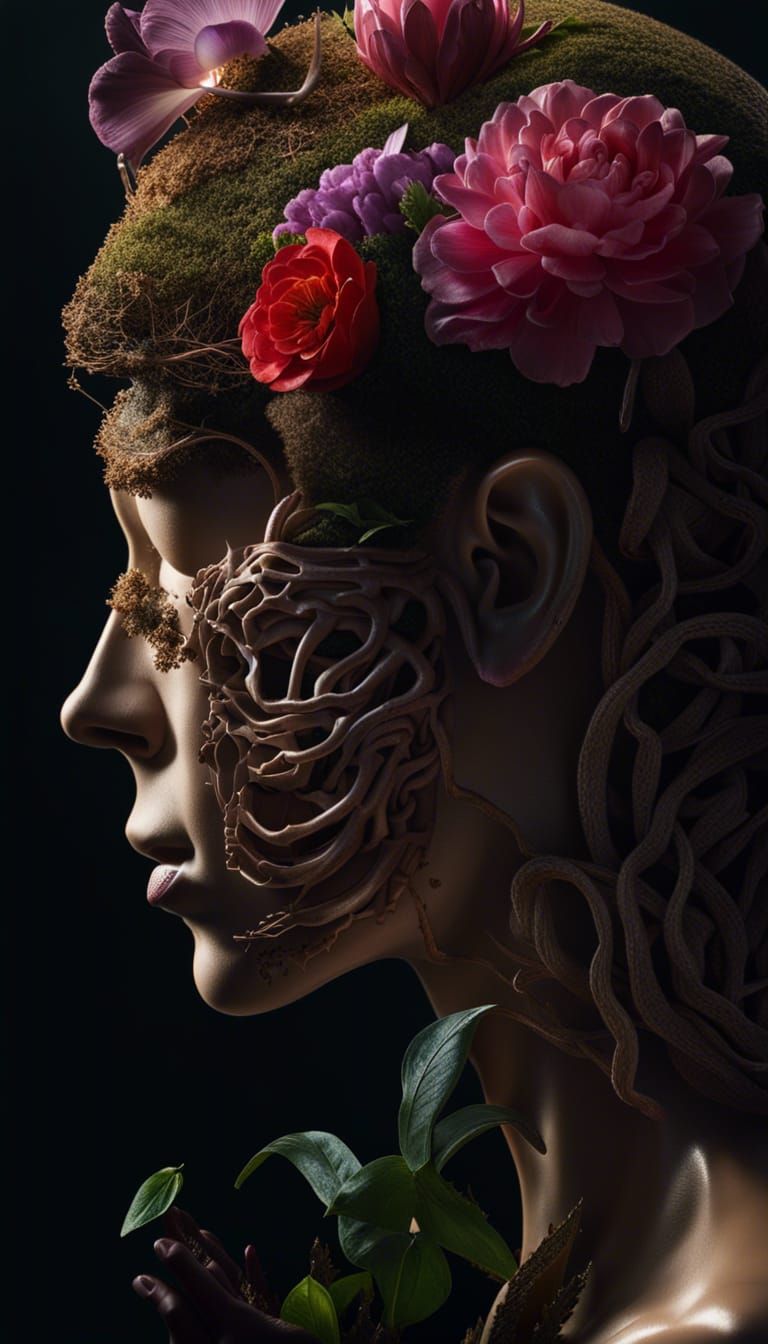The image is a vertically aligned, computer-generated artwork featuring the left profile of a woman's face. The face has a peculiar mixture of natural elements and synthetic features. The woman's eyes and mouth are closed, and her nose is normal. Instead of smooth skin on her left cheek, there is a textured pattern resembling twisted and circular worm-like fibers. Emerging from under her eye is a stem that adds to the intricate detailing. Atop her head, short green moss replaces traditional hair, interspersed with a collection of vibrant flowers. Prominently, there's a large pink flower on the upper right side and smaller clusters including red and purple flowers throughout, with larger purple petals illuminated by a light source behind them. The background is solid black, which highlights the details from top to bottom, including some green leaves with purple-tinted stems growing under her chin. The artwork gives the appearance of a statue or model, rendered with a surreal and bizarre aesthetic that blends organic and artificial elements.